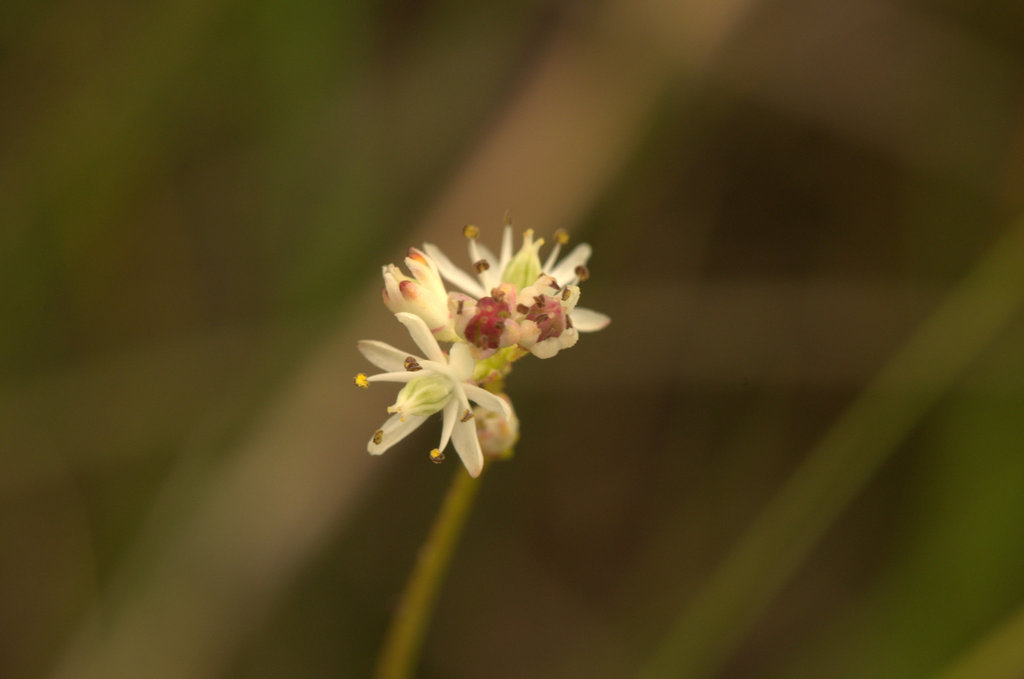This is a close-up, horizontal landscape image captured using a macro lens set at an aperture of 1.8, resulting in a striking bokeh effect that blurs the background while maintaining intricate details on the focal point—the flower buds. At the center of the image, small white flowers are prominently displayed with remarkable clarity, showing off their delicate petals and stamens. Detailed bits of pollen are visible, particularly on the red stamens in the bloom of the white flowers. The flowers are surrounded by petals that are predominantly white, though some tips exhibit shades of yellow, pink, and red. The composition features multiple stages of bloom: one flower at the bottom left in full bloom with six evenly spaced petals and five arms extending from the center ending in tiny yellow bulbs, a partially open bud, and two closed buds with maroon or pinkish-colored centers. The stem of the plant is green, contrasting against a background blurred in shades of green, light green, dark green, white, and hints of brown, accentuated by lines and an overall greenish-brown hue.